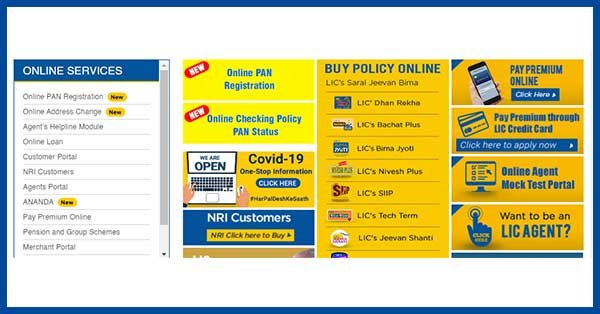The image features a detailed layout with a blue border surrounding a white interior. On the left side, there is a blue rectangle with white text that reads "Online Services." The central section lists various services in blue text, including:

- Online PAN Registration
- Online Address Change
- Agency Helpline Module
- Online Owned Customer Portal
- NRI Customer's Agency Portal
- ANANZA
- Pay Premium Online
- Pensioning Group Schemes
- Merchant Portal

Additionally, some lines of text in yellow and blue mention services like Online PAN Registration and Online Checking Policy PAN Status.

Towards the bottom, there is a red section related to COVID-19, featuring a generic laptop graphic with the text "We are open." Beside this, there is a blue-bordered white section stating "NRI Customer's."

A prominent yellow rectangle with blue text declares, "Buy Policy Online."

Other sections within the layout include various services and announcements, such as:

- Pay Online Premium
- Pay Online Premium through LIC Credit Card
- Online Agent Mock Test Portal
- Want to be an LIC agent?

The overall layout suggests it is a digital interface for an insurance company, likely providing various online services and resources for customers, agents, and NRI clients.